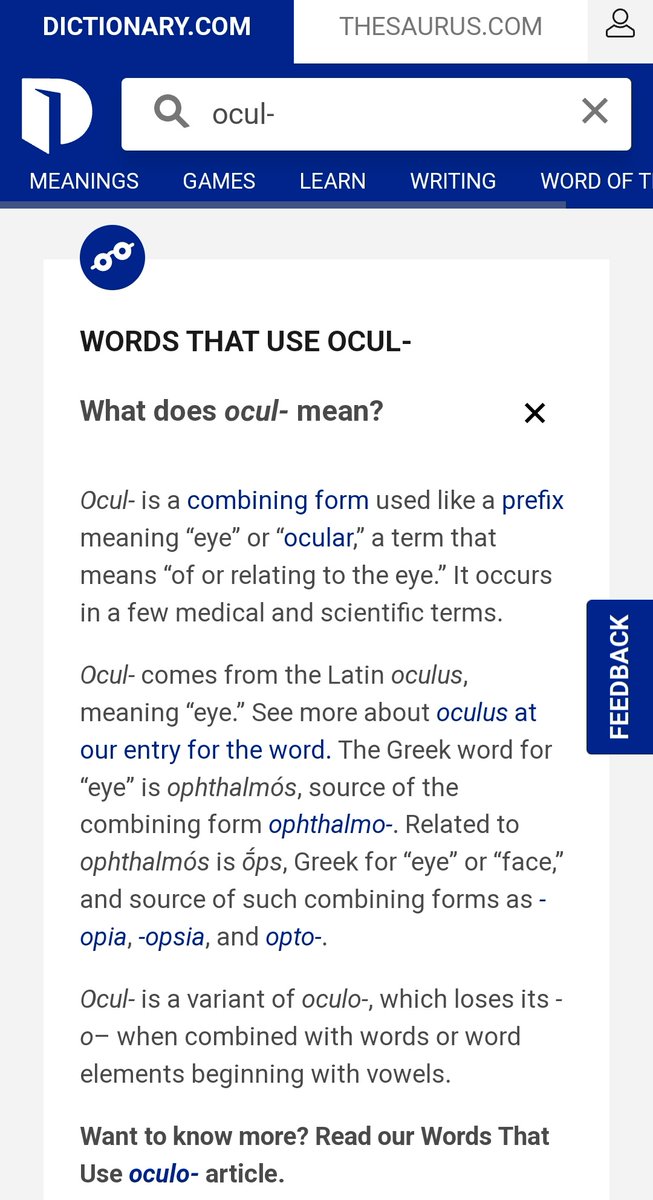The image features an interface from Dictionary.com and Thesaurus.com at the top. On the left, the blue background showcases "DICTIONARY.COM" in uppercase, while on the right, "THESAURUS.COM" is displayed on a white background. Adjacent to this is a silhouette of a person, followed by a search bar containing the letters "O-C-U-L" and a hyphen. Below the search bar, within the blue header, are navigation options labeled "MEANING," "GAMES," "LEARN," "WRITING," and "WORD OF." A blue circle with two small white circles, reminiscent of glasses, is also present.

Further down, black text introduces "Words that use O-C-U-L-." A question follows: "What does O-C-U-L- mean?" This section includes three explanatory paragraphs. The first paragraph, partly highlighted in blue text, states that "O-C-U-L-" is a combining form (in blue), used like a prefix (also in blue) meaning "eye" or "ocular" (in blue quotations). The term "ocular," highlighted in blue, is defined as relating to the eye. The explanation continues to state that it appears in medical and scientific terms. Two additional paragraphs provide further details. At the bottom, black text invites readers to "Want to know more? Read our words that use A-O-C-U-L-O- article."